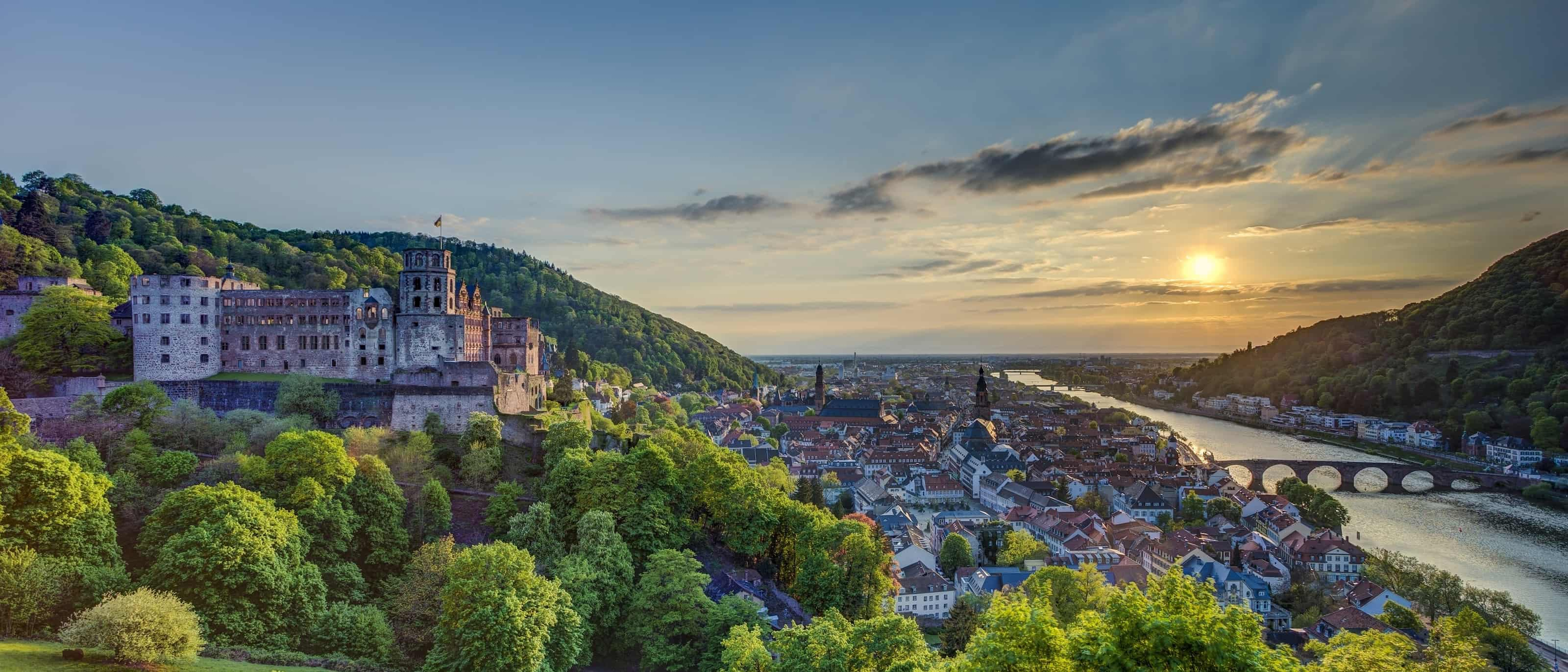The image depicts a vivid and picturesque outdoor scene, likely captured from an elevated perspective, possibly via drone. To the right, a shimmering silver river runs through the landscape, crossed by a distinct bridge. On the far right, a verdant hill, dotted with trees, adds depth to the scene. The sky above transitions from a light blue to a yellow-gray hue with scattered gray and white clouds, illuminated by the setting sun in the top right corner.

Dominating the left side of the image is a sprawling, castle-like building featuring numerous cylindrical structures, with sections of white cement and light brown walls. This structure prominently displays a flag atop one of its towers. Surrounding this architectural marvel and continuing towards the center is a cluster of houses, characterized by close proximity, white walls, and rooftops in varying shades of brown and gray.

Green trees and bushes are interspersed throughout the landscape, flourishing on hills and near residential areas, giving a sense of lushness and life. The overall clarity of the image is enhanced by the bright, natural lighting, making the details of this small city or village, with its mixture of architectural elements and natural beauty, easily discernible.